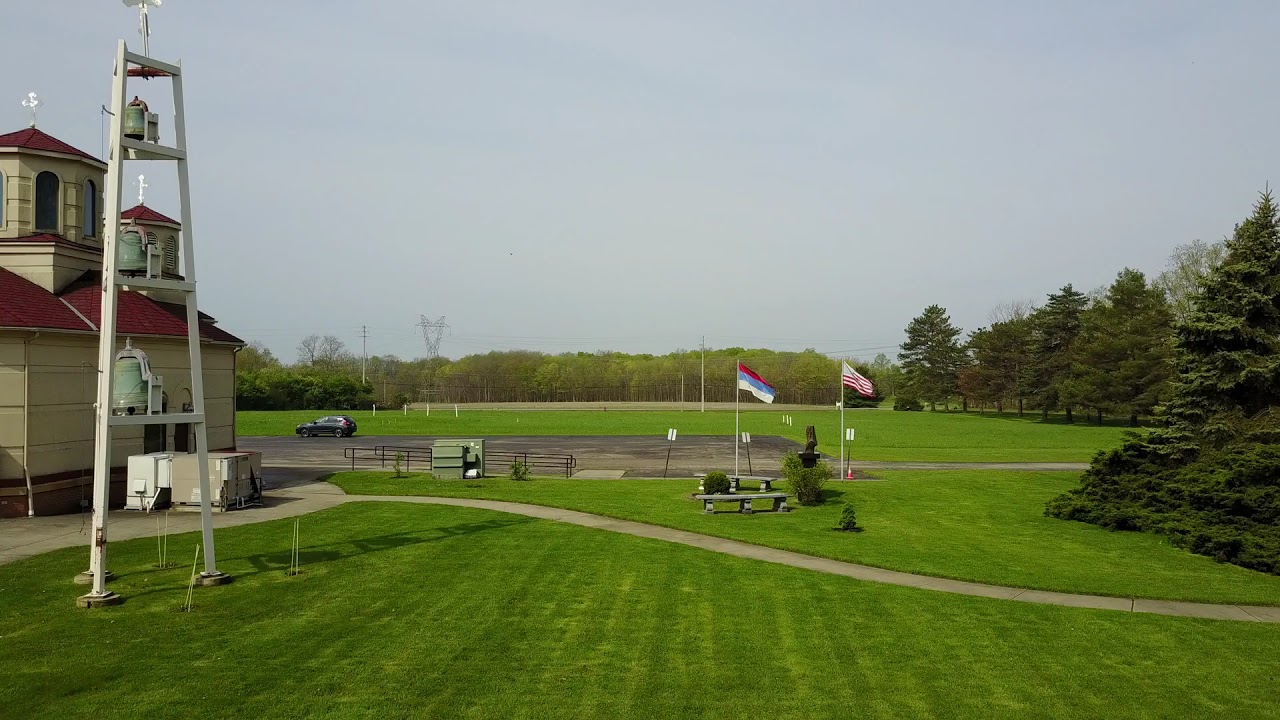The photograph captures a bright, outdoor scene with a slightly elevated view. In the foreground, a large, freshly mowed lawn occupies much of the image, complete with visible mower tracks. A long, curving sidewalk starts at the lower right corner and extends toward the left center of the image. Prominently featured on the left side is a building that appears to be a church, characterized by its tan walls and red roof. Adjacent to this building is a steel-colored tower with several bells.

In front of the church, a three-sided, ladder-shaped structure runs the height of the image. Two flagpoles stand prominently, one bearing the American flag and the other a flag with red, light blue, and white stripes. A small parking lot is centrally located in the image, and to the right of this lot, a road stretches off before disappearing behind large trees. Beyond the parking lot, the lawn extends to a fence, with a row of trees providing a natural border. Additional trees frame the scene on both the right and behind the main building, adding to the lush greenery of the setting.